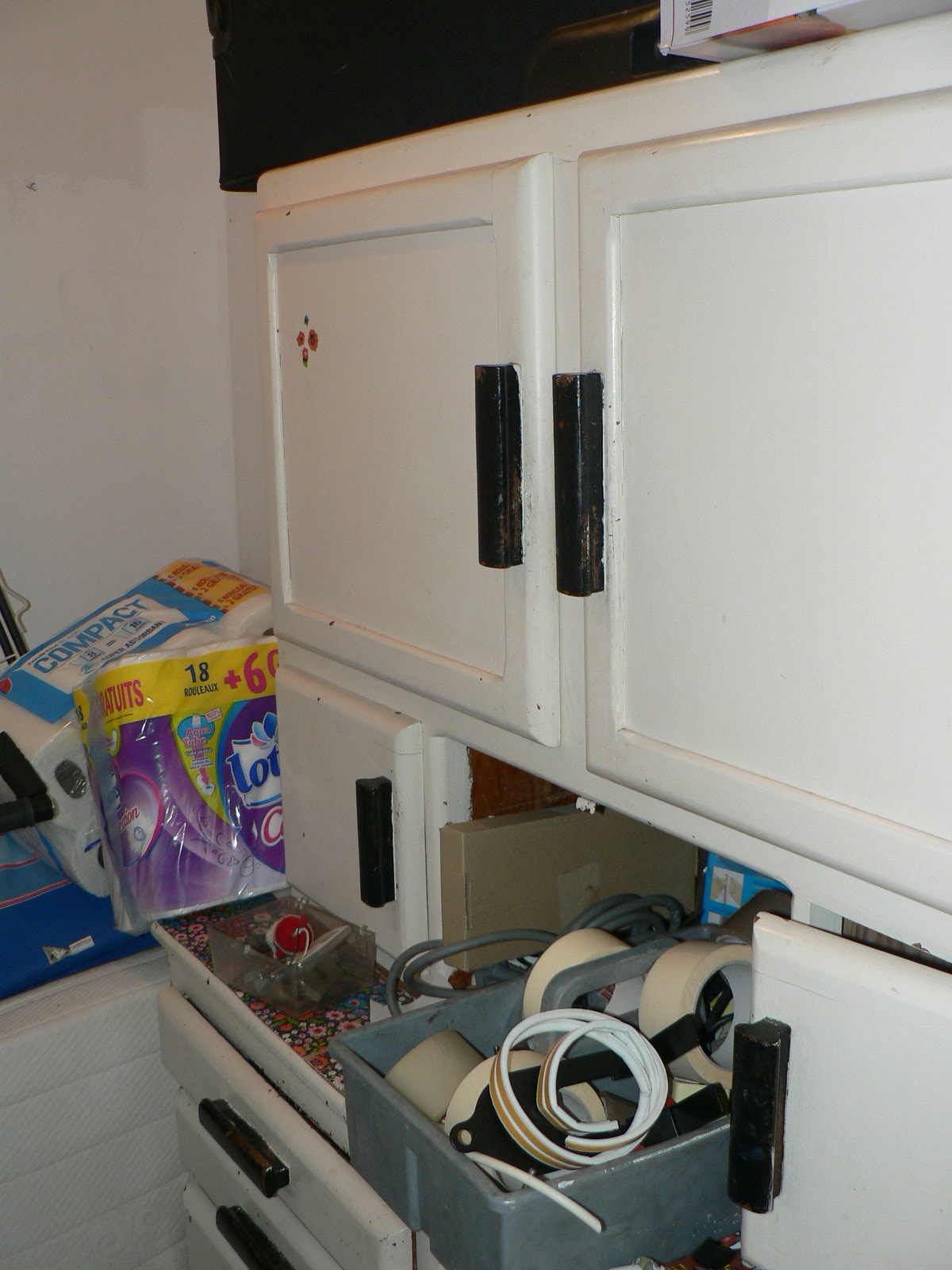The image showcases a wooden cabinet in a room, though the specific room is not identified. The cabinet is painted white, albeit with visible imperfections, suggesting a somewhat rushed or amateur paint job. The cabinet doors, which include painted handles, do not all close properly; some are partially opened or propped ajar. A red decal adorns one of the cabinet doors, adding a pop of color. Along the top edge of the cabinet runs a brown border, contrasting with the predominantly white surface.

To the left of the cabinet, there's a white-painted brick counter. The interior of the cabinet reveals unfinished wood, particularly noticeable where items are pulled out, exposing the boundaries of the white paint. Within the cabinet, there is a silver box filled with tape and wires.

One of the cabinet doors or drawers features an unsightly laminate pattern. Various household items are visible in the background, including rolls of toilet paper or possibly paper towels—distinguishable by their different colored plastic wrappings, one purple and one blue.

The white wall behind the cabinet has a visibly uneven paint job, characterized by slightly different shades where the paint seems to have been applied inconsistently, perhaps not reaching the full height with the roller or brush.

This detailed description provides a vivid visual of the scene’s elements and their conditions.